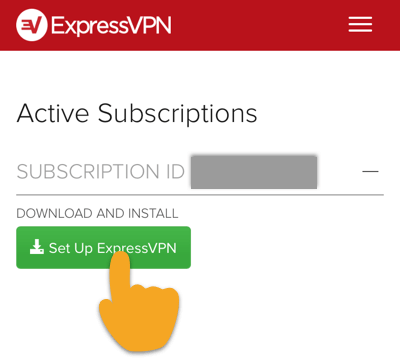The image is a portrait-oriented screenshot or photograph of a webpage, likely from the ExpressVPN website or its software interface. 

At the top of the page, there is a distinctive red border. Within this border, the "ExpressVPN" branding is displayed prominently in white font, accompanied by the ExpressVPN logo on the left— a white circle featuring a stylized 'V' with lines extending from its left side. To the right within this red border is a white hamburger menu icon, indicating additional menu options.

Below this header, the content area begins with ample white space, leading to a section header titled "Active Subscriptions" in black text. Directly beneath this is the label "Subscription ID" in gray text, followed by a gray box that obscures specific subscription information, likely for privacy reasons.

Following this, there is a thin gray line that serves as a separator. Below this line, more white space introduces a section labeled "Download and Install." Centrally positioned in this section is a prominent green rectangular button with white text that reads "Set up ExpressVPN," accompanied by a download icon to the right.

Adding a guiding visual cue, a hand emoji—depicted as a right hand with the index finger pointing— is overlaid on the green button. The finger specifically points at the letters 'P' and 'R' in "Express," clearly indicating to users that they should click this button to proceed with setting up and launching ExpressVPN. 

This detailed composition and deployment of visual aids aim to guide users through the process of activating and installing the VPN software.